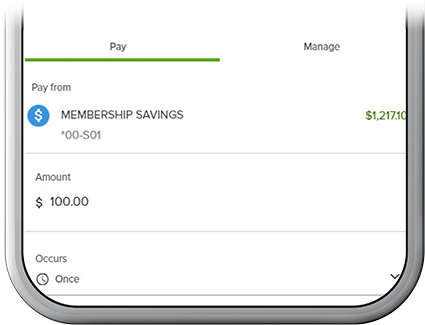This animated screenshot showcases the bottom one-third of a smartphone interface against a light gray border. The main screen has a clean white background and displays two options at the top: "Pay" and "Manage." The "Pay" option is selected, indicated by a green bar beneath it. The interface is divided into three distinct sections:

1. **Pay From**:
   - A blue circle with a dollar sign icon.
   - To its right, the text "Members to Membership Savings" is written in capital letters.
   - Adjacent to this, highlighted in green, it shows "$1,217.10."
   - Below this, there is an identifier: "Member Savings *00-S01."

2. **Amount**:
   - Displays a dollar sign followed by "$100.00."

3. **Occurs**:
   - Features a clock icon alongside the word "Once."
   - Includes a caret symbol, suggesting a drop-down menu for frequency options.

This detailed layout provides clear and organized information about payment options, amount, and frequency, ensuring user-friendly navigation and understanding.